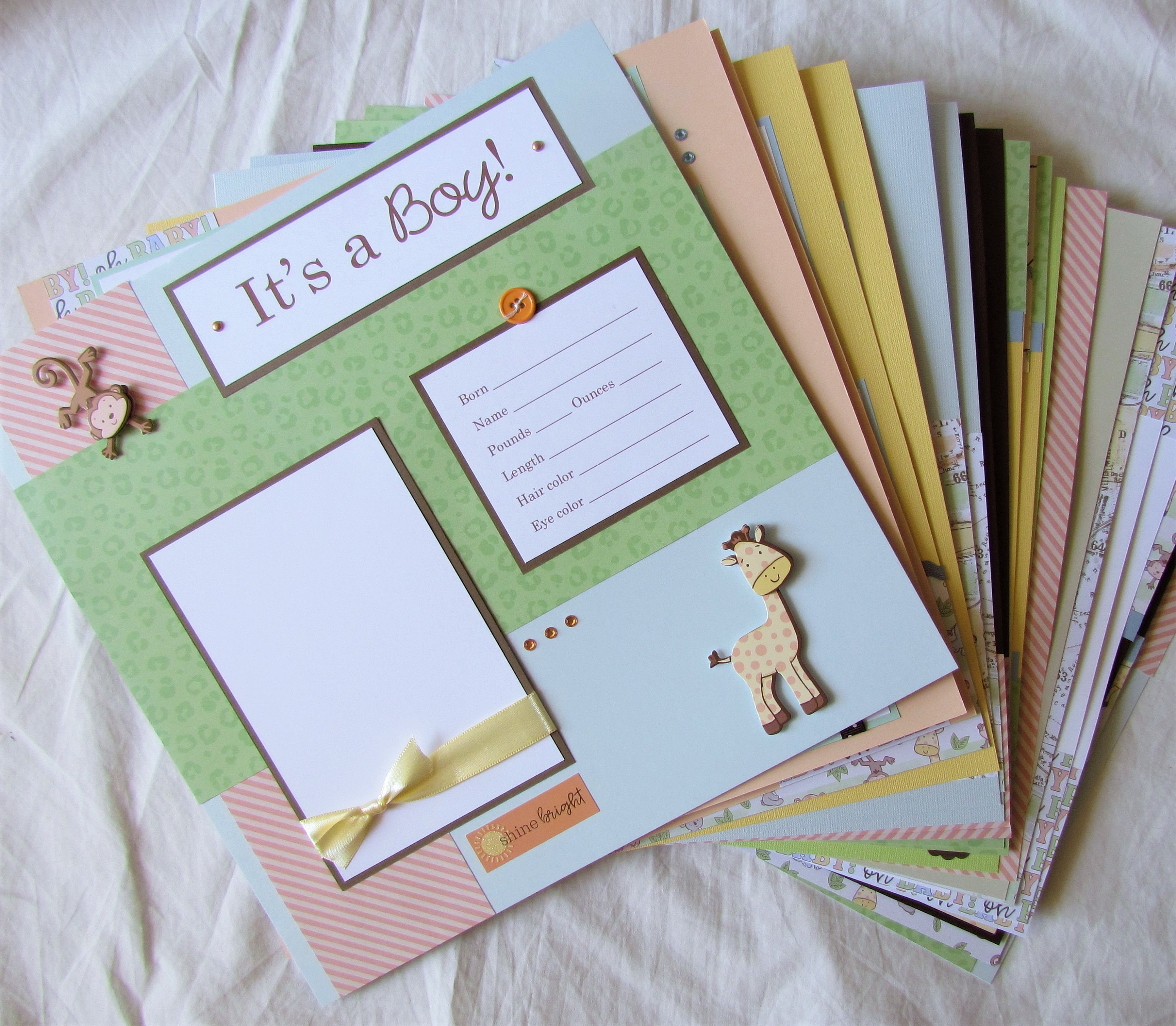The image depicts a fanned-out arrangement of scrapbook pages meticulously laid on a creased, off-white sheet. Dominating the scene is the topmost page, framed by an olive rectangle that contains the text "It's a boy!" in a white rectangle. This page also features various embellishments, including a smiling, downward-facing 3D monkey figure at the top left and a similar 3D giraffe figure at the bottom right. A sticker towards the bottom left reads "Shine bright" and is adorned with a sun illustration. The central scrapbook page sports a blue background with a pink diagonal stripe pattern. Additional details include a white label with a brown border that reads "Born" followed by lines for filling in details about the baby's birth, another label tied with a yellow ribbon, and a sewn-on orange button. Together, these elements create a vibrant and textured homage to a newborn's arrival.